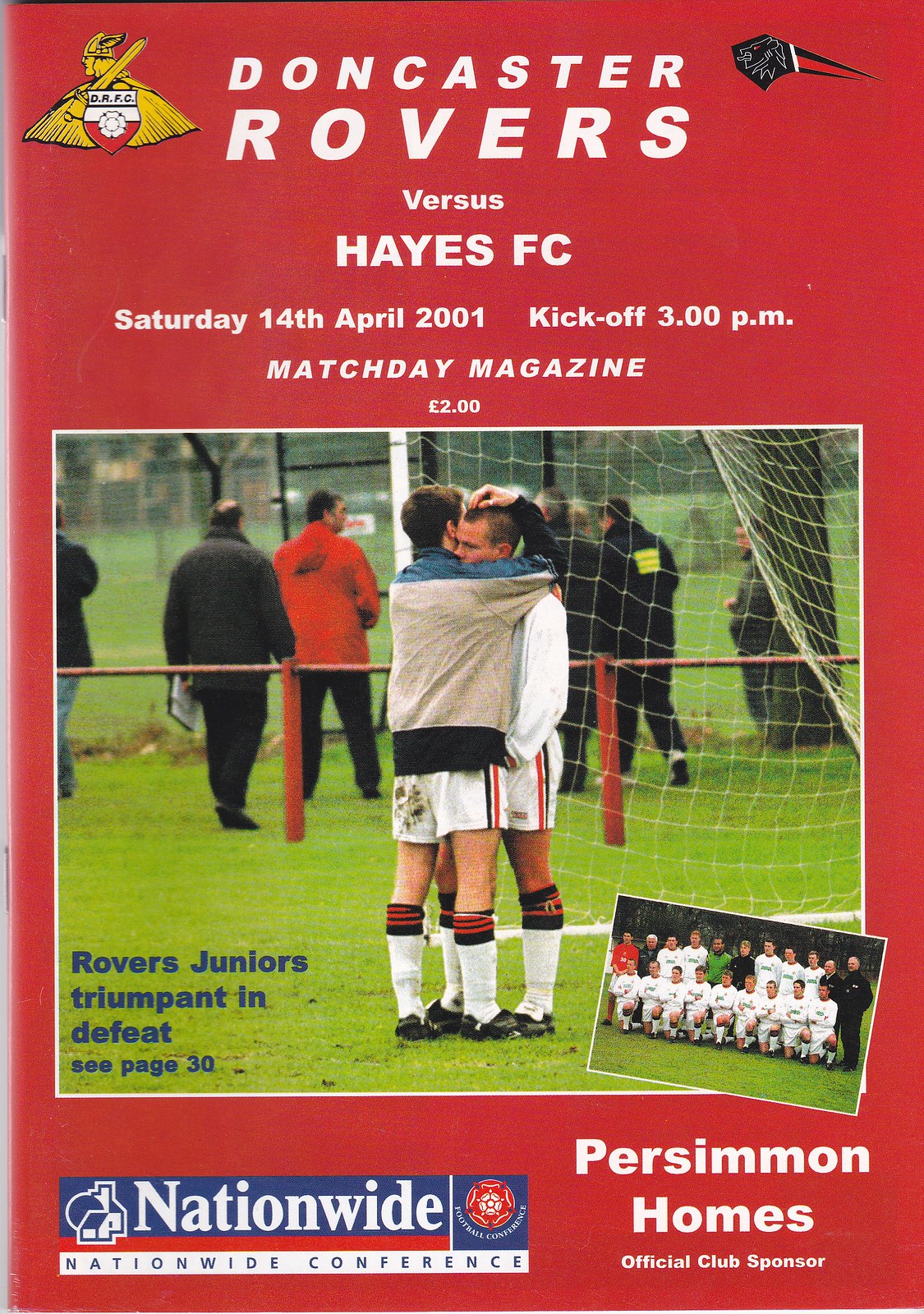This image is a rectangular flyer, approximately six inches tall by three to four inches wide, resembling the front cover of an old magazine with staple marks on the left-hand side. The background is a striking red. At the top, in white print, it announces: "Doncaster Rovers versus Hayes FC, Saturday, 14th April 2001, Kickoff 3 p.m." 

An eye-catching gold insignia featuring a Viking with a sword and a red and white shield occupies the upper left corner, accompanied by the abbreviation "DRFC." Directly below, it specifies: "Match Day Magazine, 2 pounds." 

Visible at the bottom center, there's a photograph displaying two soccer players in white shorts with red and black striped uniforms, embracing in front of a goalpost with white netting. Alongside this, in blue font, is the caption: "Rovers Juniors Triumphant in Defeat. See page 30." 

In the lower right corner, the image includes a smaller picture of the entire team dressed in their soccer gear. The flyer is sponsored by "Nationwide Conference," featured in a blue font at the footer, and "Persimmon Homes," marked as the official club sponsor in white print. The overall design captures the essence of an English football match advertisement from 2001.